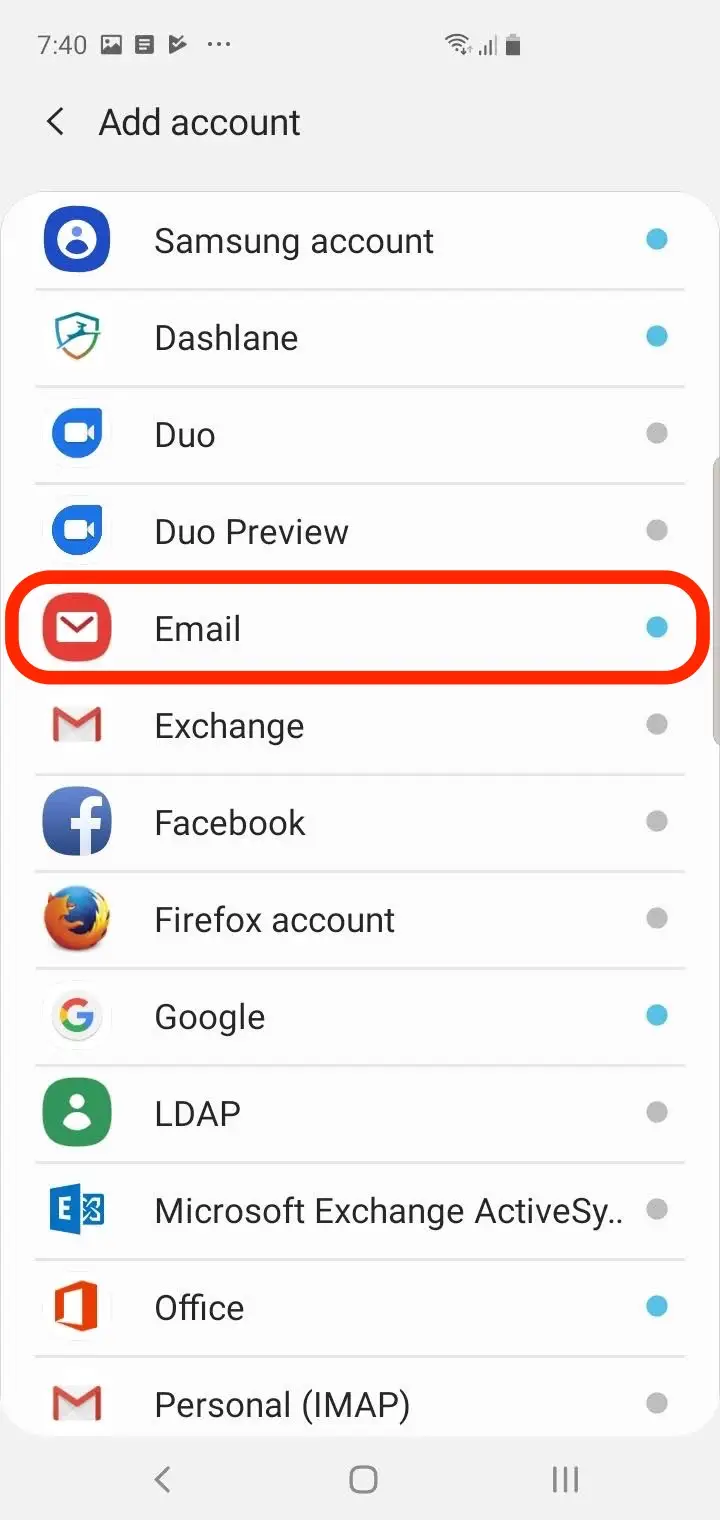The image displays a smartphone screen showcasing various account icons and statuses in the "Ad Account" section. At the top left, "Ad Account" is written in black text, and directly underneath it is "Samsung Account" accompanied by a blue dot on the right. On the left, there is a blue circular icon containing some white details.

Below the "Samsung Account" is a section marked by a dashed line. To the left, there is a green icon with an image of a springbok, also accompanied by a blue dot on the right. Further below, you'll find the "Duo" account, represented by a blue icon featuring a white video camera. The corresponding dot on the right side is grey, indicating a "Duo Preview" label with the same icon.

Next is the "Email" account, indicated by a red envelope icon on the left. The blue dot on the right shows its active status. The "Exchange" account trails, marked by a white envelope with an "M" and a grey dot on the right. 

The sequence continues with the "Facebook" account, characterized by a blue icon with a white "F" and a grey dot. The "Firefox Account" follows, using a blue icon with a yellow fox; its dot is also grey.

The list also includes:
- "Google Account": This icon is distinguished by the multicolored "G" in red, yellow, green, and blue, and features a blue dot.
- "LATPro": Identified by a green icon and a grey dot.
- "Microsoft Exchange ActiveSync": Marked by a grey dot.
- "Office": Represented by an orange icon and a blue dot.
- "Personal IMAP": Displayed with a Gmail icon and a grey dot.